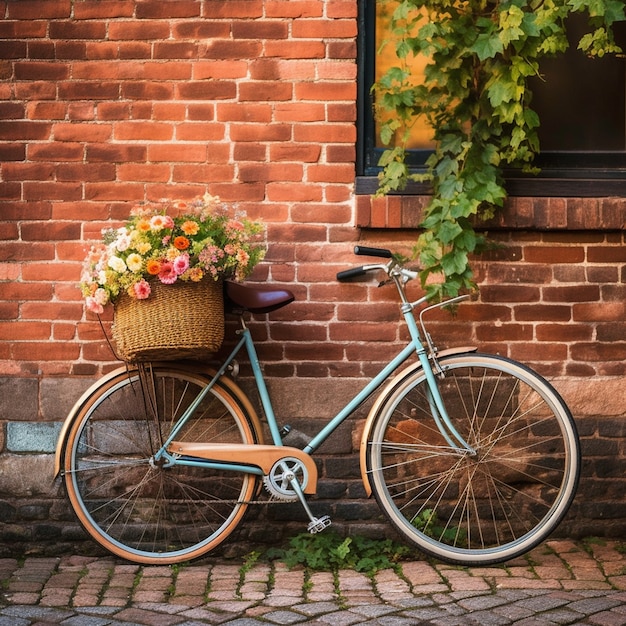This image captures a tranquil scene featuring a vintage-style, teal bicycle leaning against a well-maintained red brick building. The bicycle, which appears to be a women's model with a brown leather seat and black handlebars, exudes a nostalgic charm. It has tan fenders and a large tan woven basket overflowing with colorful flowers, including shades of pink, orange, yellow, and white, with some greenery interspersed. The bike's tires are banded in light brown and white, and a faintly rusted chain can be seen. The rear tire supports the heavily laden basket, adding to the bike's quaint appearance.

The backdrop of the scene is a rustic brick wall composed of handmade bricks in varying shades of red. A black-framed window on the upper right corner of the image is partially shrouded by trailing ivy, which adds a touch of nature to the man-made structure. The window reflects a golden sunlight, suggesting a warm, sunny day. The ground beneath the bicycle consists of a cobblestone pathway with some greenery peeking through the gaps between the stones. The overall setting has a soft, golden glow, either due to the natural sunlight or a photographic filter, giving the image a serene and idyllic atmosphere.